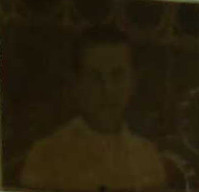This image is a very small, square, low-resolution portrait of an individual with indistinct facial features. The person, whose gender is indistinguishable, has a neutral expression and wears a light-colored, short-sleeve shirt. They have short black hair and dark eyebrows, and appear to be Caucasian. The overall tone of the photo is very dark, almost black and white but with a subtle brown or greenish hue, suggesting an aged photograph from perhaps the early 1900s. Only the head, shoulders, and upper chest of the person are visible, with no facial hair. The background is predominantly black and features indistinct patterns, possibly vertical lines and circles, and might have some leaves or plant elements on the right side.